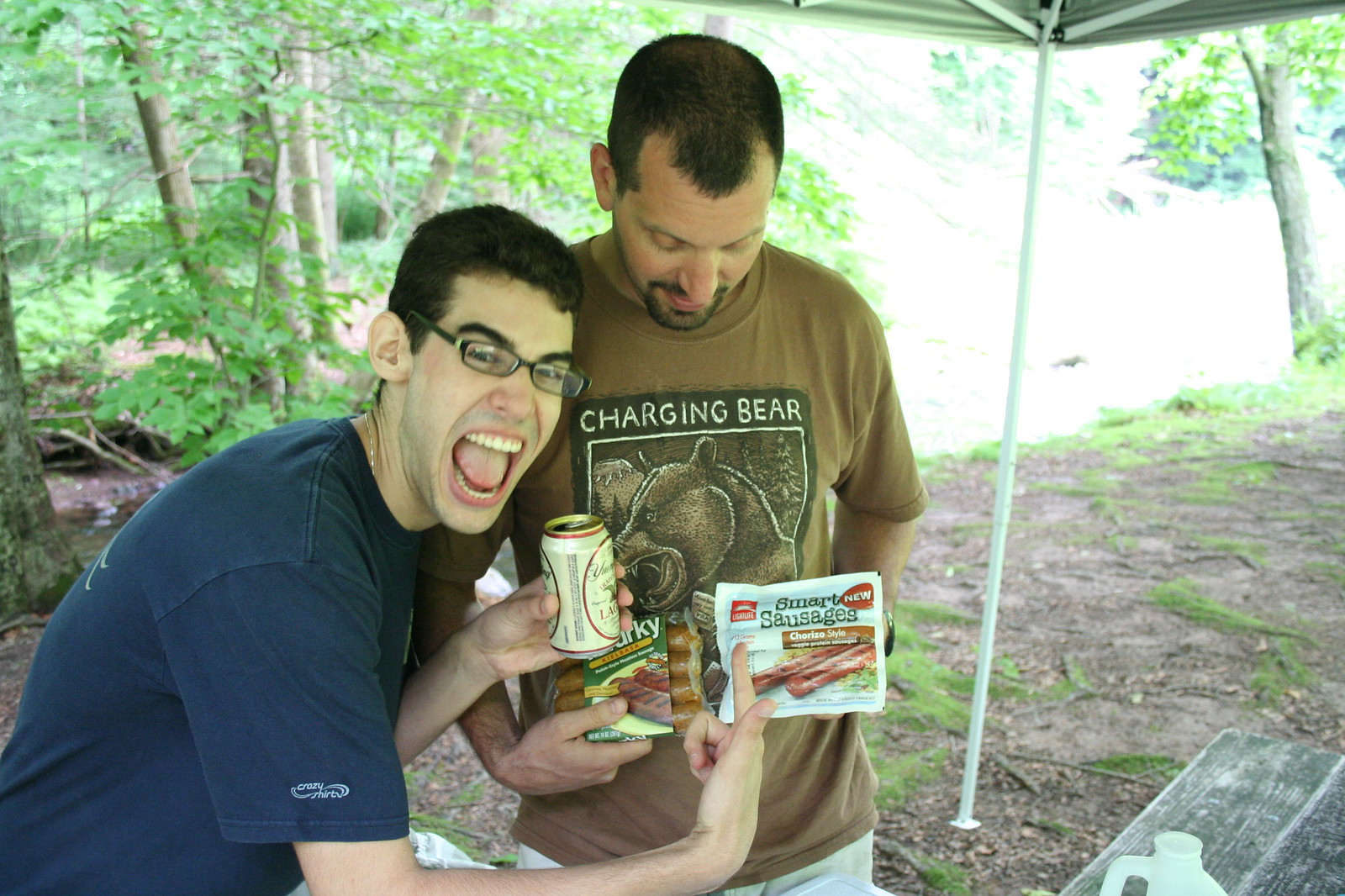The photograph captures two men enjoying an outdoor setting, possibly a campsite or picnic area, under a steel frame canopy with a tarp roof. The man on the left, who has short black hair and wears black-framed glasses, is energetically interacting with the camera with his mouth open as if shouting. He's dressed in a blue t-shirt and holds a can of Yingling beer in one hand, while in the other, he presents a package of Smart Sausages, chorizo style. The man on the right is standing more centrally in the frame and has short black hair with a mustache-goatee combination. He sports a brown t-shirt that features the text "Charging Bear" along with a cartoon image of a bear. This man holds a pack of turkey sausages. They are positioned near a picnic table, partially visible at the right edge of the frame, which holds a white plastic jug likely containing water. The background is lush with greenery, showcasing a forest and a river, with sunlight filtering through the leaves, enriching the scene with a vibrant natural ambiance.